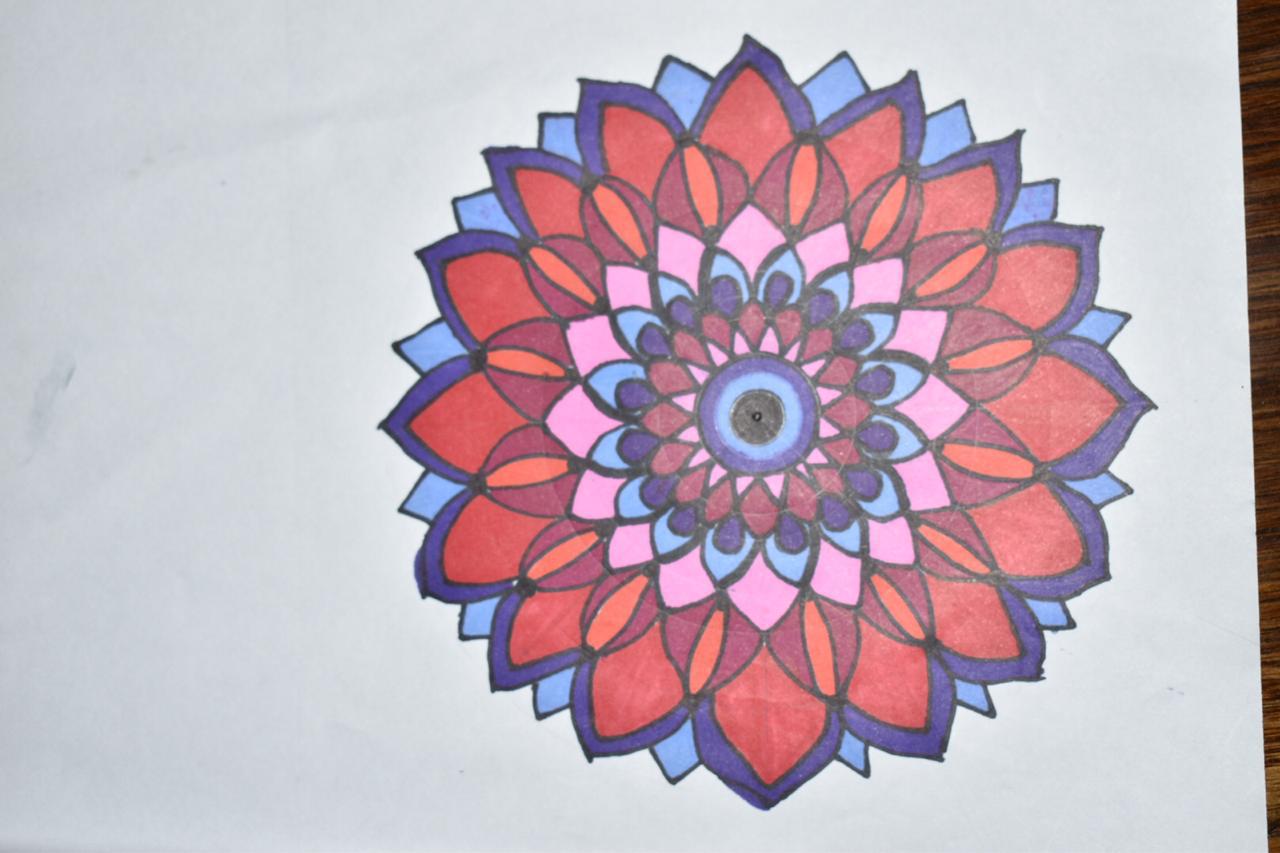This image is a photograph of a detailed, hand-drawn, colorful illustration that seems to represent an abstract flower, though not one found in nature. The drawing features multiple concentric layers of geometric shapes resembling petals, with both triangular and rounded designs. The center of the flower is black, surrounded by a ring of light blue, then intense dark blue before transitioning into layers of petals. These petals exhibit a rich array of colors including pink, red, dark purple, orange, and multiple shades of both blue and purple. As the illustration radiates outward, the petals vary in size and pattern, incorporating intricate combinations such as light blue encompassing dark blue teardrops and purple petals with lighter pink bases. The entire illustration is outlined in what appears to be black pen or felt tip. The drawing is photographed against a dark brown wooden surface, visible as a thin vertical strip along the right edge where the paper does not fully cover the background.